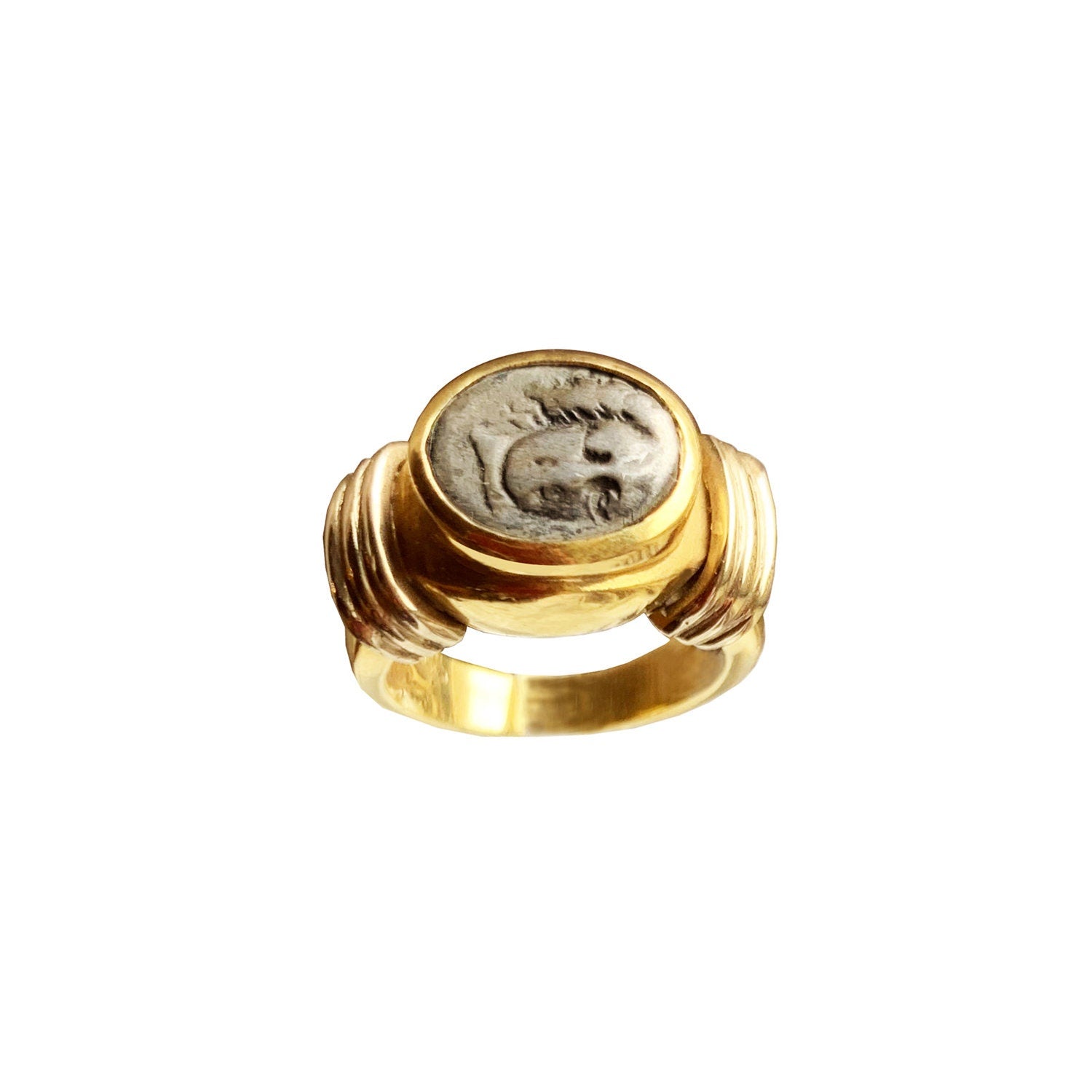The image showcases a gold ring set against a pure white background, devoid of any drop shadow, suggesting it has been edited for clarity. Viewed from a top-down perspective, the ring features a central oval section where an old and worn-looking male face is carved in a dull silver-esque metal, reminiscent of an ancient coin. Encircling this central face are three shiny and well-polished gold bands on either side, making up a total of six rings around the main structure. The ring's detailed and seemingly historical appearance evokes curiosity about its origins and craftsmanship.